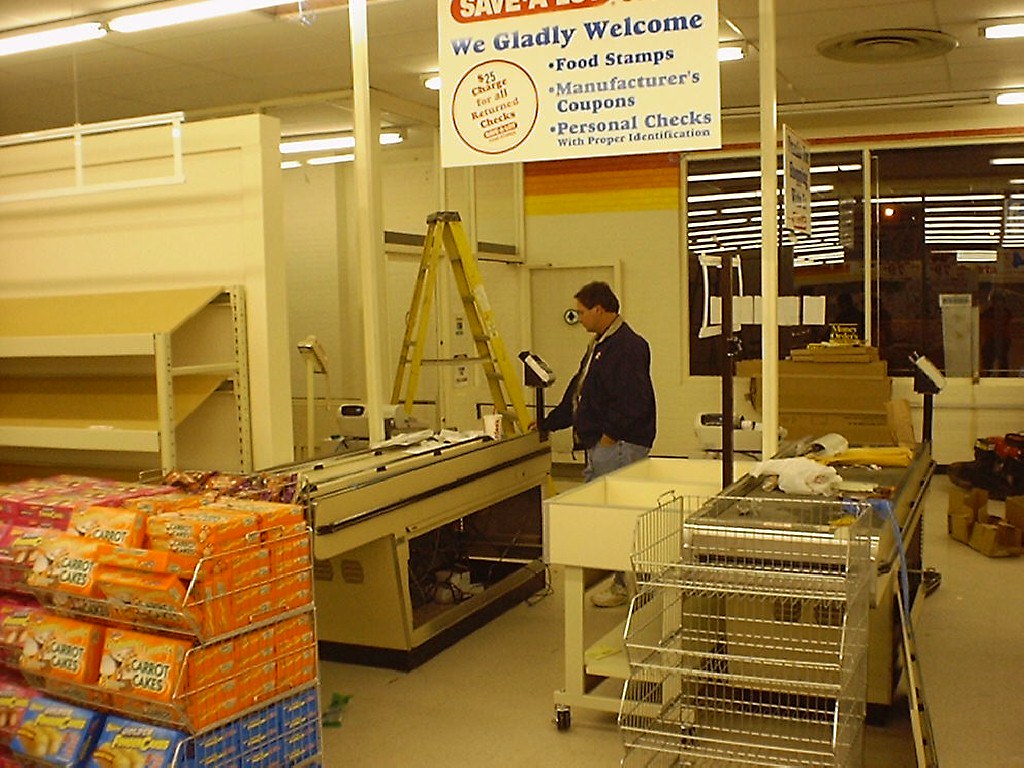In this detailed photograph taken during a grocery store remodel, the scene is set with various elements that illustrate the transformation in progress. In the front left-hand corner, there are a few shelves stocked with prepackaged food items, including distinctly visible orange boxes labeled "carrot cakes." Adjacent to these are some red and blue boxes, the labels of which are not clearly readable. Near these food items, you can see white metal fixtures featuring tan-colored wood shelves, which are currently empty and angled slantwise.

A man dressed in a blue jacket and blue jeans stands prominently in the center of the image, positioned beside a yellow ladder and in front of what looks like a conveyor belt typically found at the checkout area. To his immediate right, there's a white rolling table. In front of another conveyor belt, a silver, empty three-tiered rack is visible. Both conveyor belts are cluttered with various loose items scattered around. The background reveals tinted dark-colored windows, adding to the overall dim ambiance of the space.

Above the scene, a sign hangs that reads: "We gladly welcome food stamps, manufacturer coupons, personal checks with proper identification," indicating the store's commitment to various payment methods. The entire setting evokes the industrious and somewhat chaotic nature of a store amidst its remodeling phase.